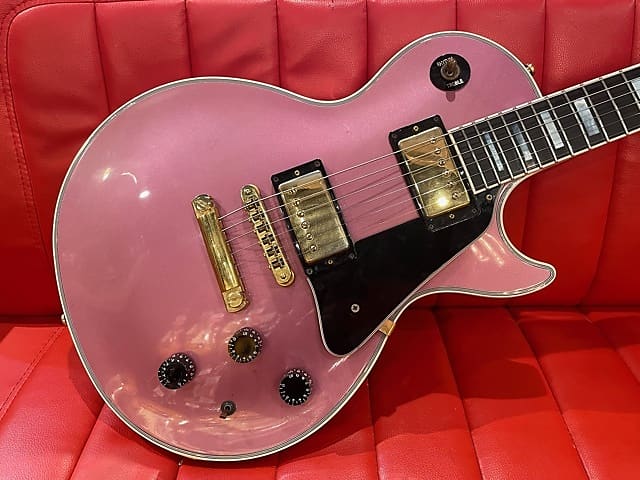This indoor image features a retro-styled electric guitar prominently displayed on a tufted, red leather couch. The guitar boasts a vibrant pink body with a smooth, rounded design reminiscent of 1950s aesthetics. Highlighting its vintage charm, the guitar is equipped with gold-colored pickups and string fasteners. It also features a black pickguard and a black neck adorned with mother-of-pearl inlays. The positioning of the guitar is such that it is centered on the red couch, with its base angled towards the top right corner of the image. The overall color palette includes pink, black, red, white, and gold tones, enhancing the classic look of the scene.